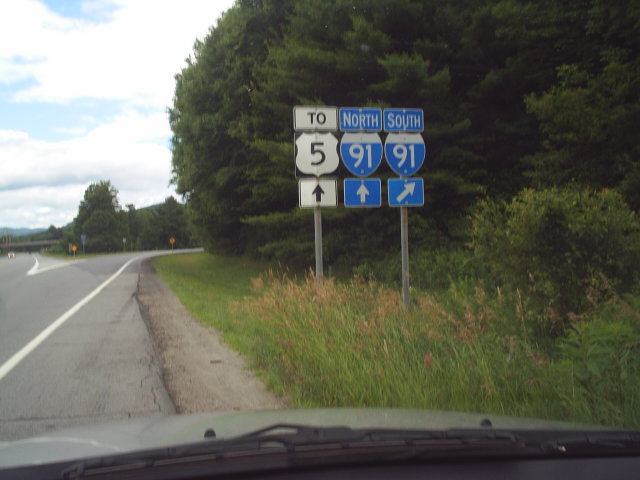This photograph, taken from inside a stationary car pulled over on the shoulder of the road, captures a scene where the roadway inclines and forks off both to the right and left. Multiple traffic and street signs are prominently displayed on two poles. The first pole has a white sign indicating "25" with an arrow pointing straight. Next to it, a sign points straight ahead, labeled "North to Interstate 91," and another sign points to the right, marked "South 91." A vehicle is approaching from the left split of the road, adding a dynamic element to the scene. Yellow cautionary signs are visible ahead along the right curve, providing important road information and enhancing the depth and detail of the image.